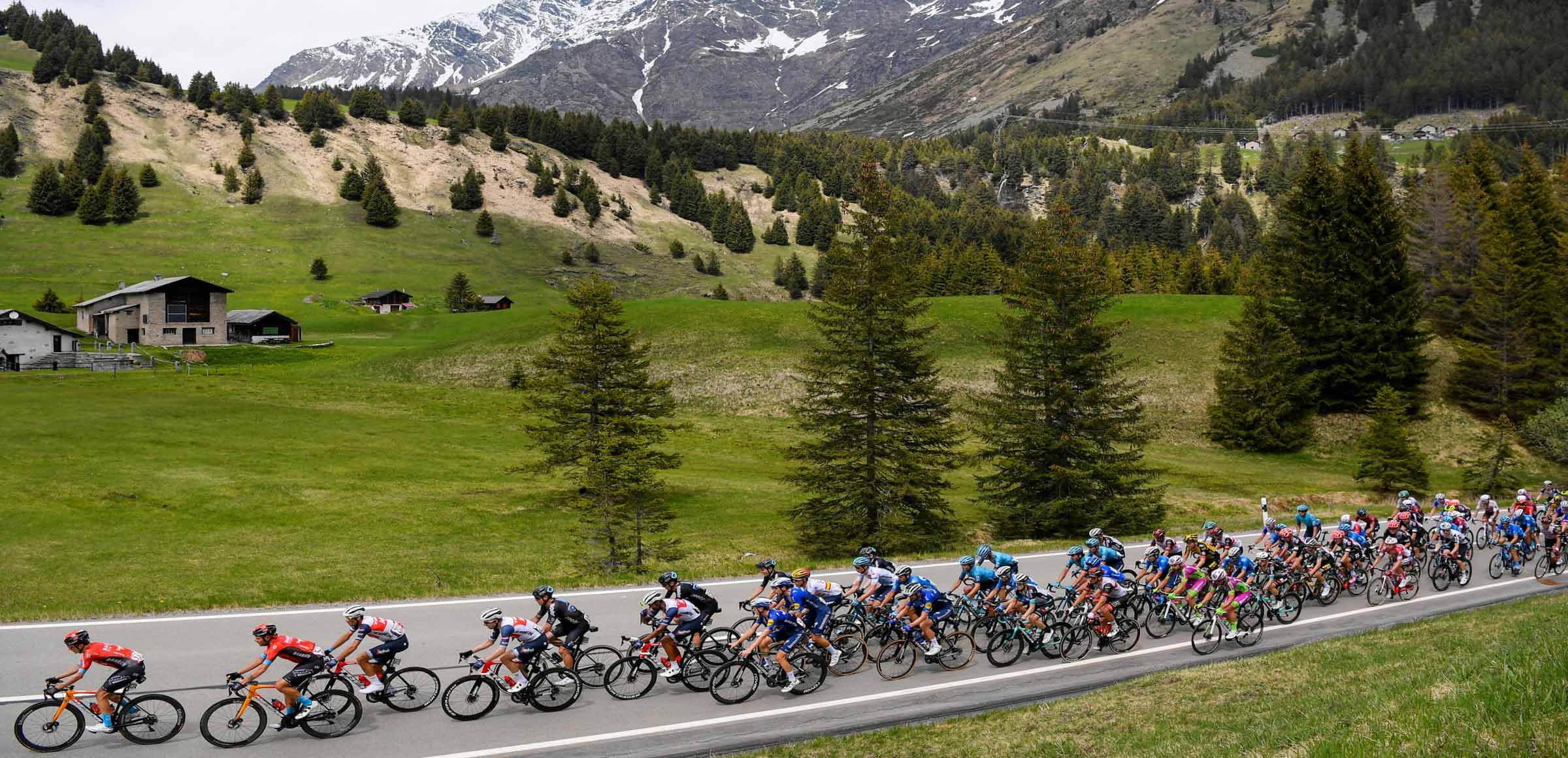This wide-angle aerial view captures a bustling bike marathon winding through a picturesque mountainside. Hundreds of cyclists, donned in colorful tight-fitting uniforms and helmets, race down the left lane of a two-lane, light gray asphalt road marked with solid white edges and dashed center lines. The right lane remains empty as the riders stretch from left to right across the frame, their individual and grouped formations varying.

In the foreground, the photograph is taken from a green and light brown grassy hill, visible in the bottom right corner. Beyond the road lies an expansive, lush green field dotted with evergreen trees. To the left, nestled in the midst of this field, stands a cluster of buildings: a beige stone house with a sloping gray roof and two smaller attachments, and a white house with a green roof.

The backdrop reveals a stunning mountain range, featuring rolling hills covered in a mix of dark green pines and patches of light brown dirt. Farther back, towering snow-capped mountains dominate the horizon, adding depth and majesty to the scene. The entire tableau combines natural beauty and athletic vigor, capturing the essence of an outdoor mountain bike race.